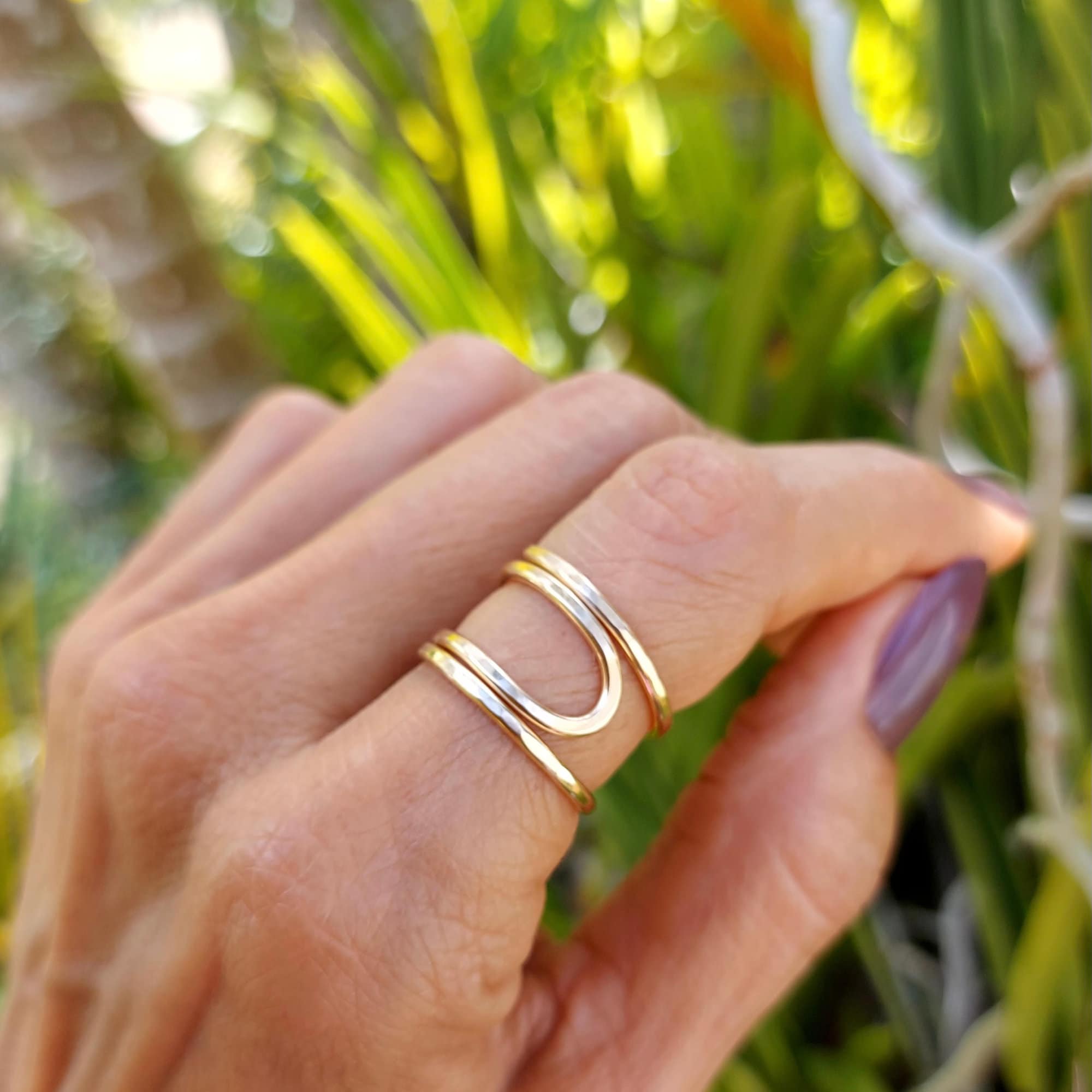This detailed image centers on an elderly person's hand making a pinching gesture. The hand appears slender, with visible bones and veins, suggesting age. The person's fingernails are well-manicured, painted a light purple shade, and adorned with some artificial, pointy nails. The main focus of the image is a thin, reflective, golden ring on their index finger. This ring has a unique design, featuring three intertwined layers that curve into each other, forming a somewhat oval shape. The background, slightly blurred, appears vibrant and green, likely an outdoor setting with elements of a garden, forest, or farm. Visible are various green plants, vines, leaves, and a tree trunk in the top left corner, creating a serene, natural backdrop for the hand.